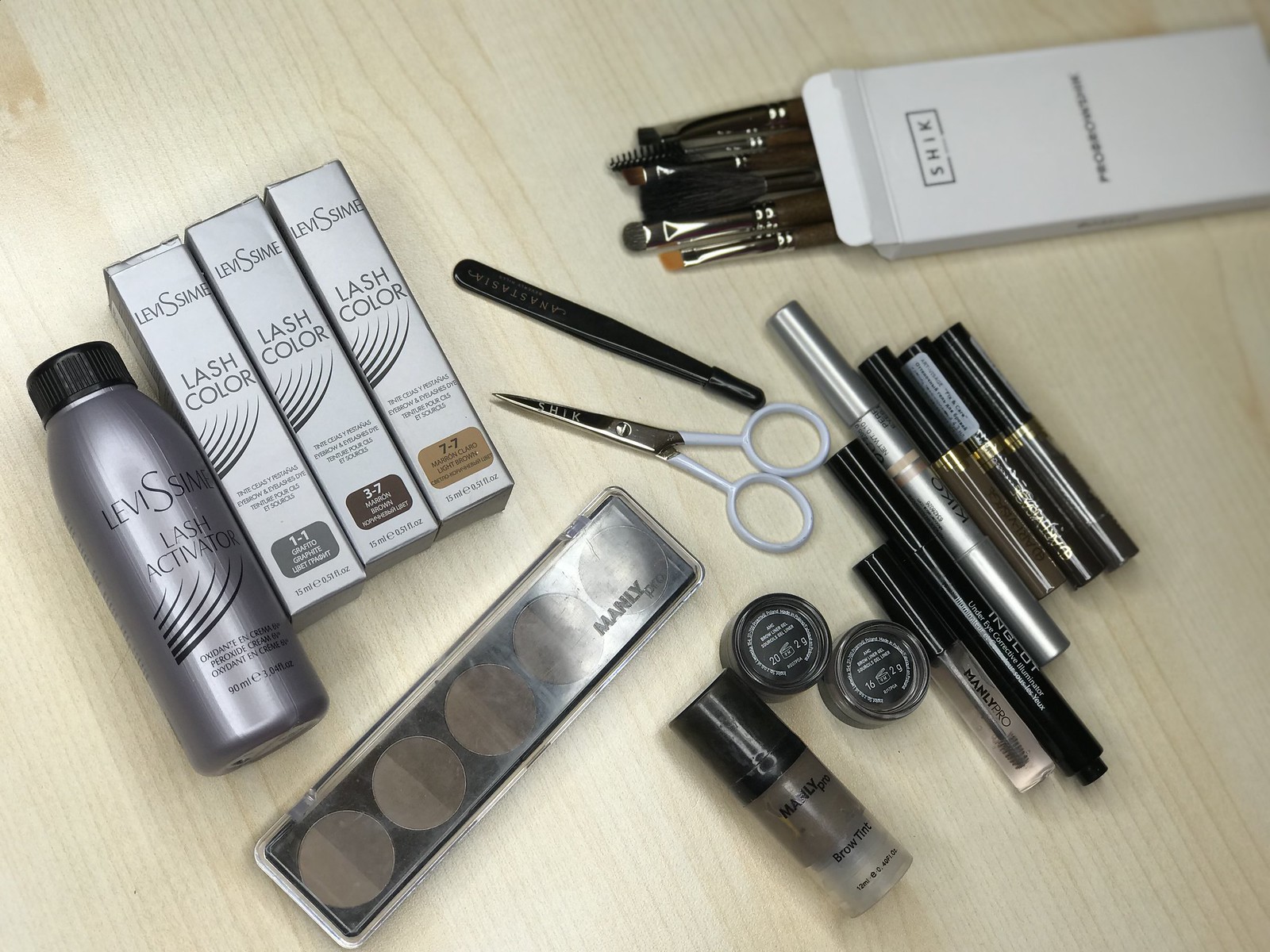On a light brown wooden table, an array of makeup products is meticulously arranged. To the left, a gray bottle with a black cap labeled "LeviSsIm Sign Lash Activator" stands prominently, featuring an illustration of eyelashes. The bottle contains 90 milliliters of product. Adjacent to it are three small packages in varying shades: Graphite, Brown, and Light Brown. Each reads "LeviSsIm Sign Lash Color," with the text available in Spanish and French.

An eyeshadow palette labeled "Manly Pro" displays a gradient of beige to dark brown hues nearby. A pair of small white-handled scissors with silver blades and a set of black tweezers are also present. A white box marked "Schick" holds an assortment of small makeup brushes, presumably designed for eye makeup application.

Also visible are two small bottles of brow tint marked "Manly Pro." Lined up alongside are six tubes of makeup: a clear "Manly Pro" tube, an all-black "Inglot" tube, a silver tube from the Spanish brand "Kiko," a brown tube with an unreadable label, and two additional black tubes.

The assortment collectively suggests a focus on eye makeup, featuring products for lashes, eyebrows, and eye shadows, complemented by the necessary tools for precision application.